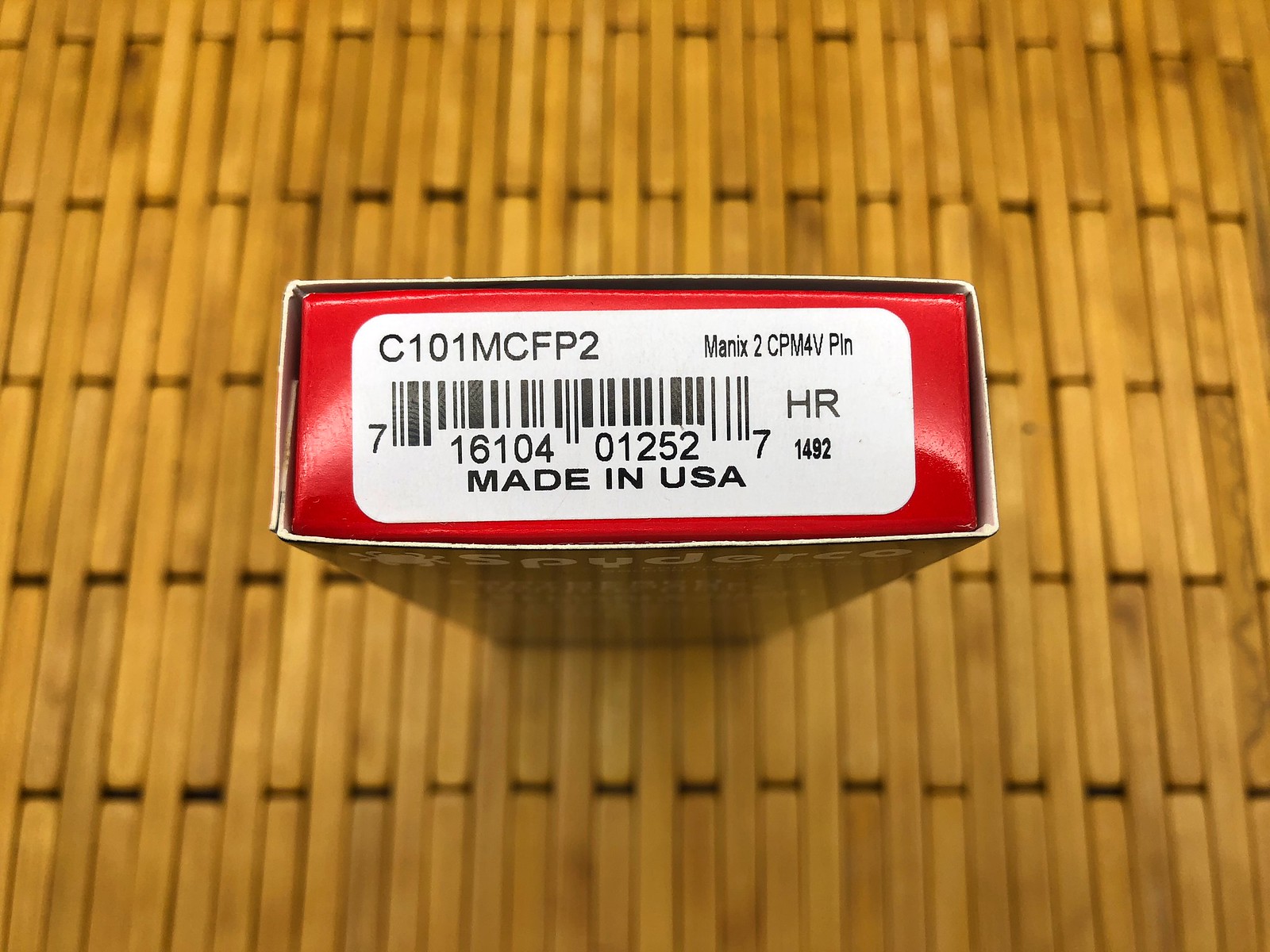A large package of classic wooden clothespins is displayed prominently, featuring a red label with white interior. The label bears black alphanumeric text reading "C-101MCFP2MNX2CPM4VPIN" alongside the words "Made in the USA." These clothespins consist of two pieces of wood held together by a spring mechanism, allowing the user to press the bottom to open the top and securely clip them onto clothes and a clothesline. The packaging also includes a barcode for scanning.